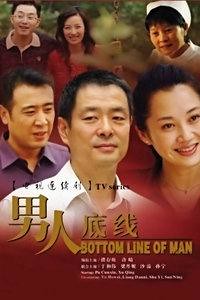The image appears to be an advertisement for a movie or series, prominently featuring six people of Asian descent against an outdoor backdrop that resembles a forest or garden with visible foliage. The advertisement is adorned with a mix of colors, including white, red, green, brown, and yellow.

The six individuals are arranged in two distinct rows. In the upper row, on the left side, there is a man with glasses in a polo shirt who is laughing or smiling with his mouth open. Next to him, towards the center, is a lady in a red outfit with long dark hair. On the far right of the upper row, a woman wearing a white cap—likely resembling a nurse's cap—and a white top can be seen. She appears to be the background character dressed as a maid.

In the center row, there are three main characters. Centered is a man with a white collared shirt, dark hair, who is looking down to the left with a slight smile on his face. To his left stands another man in a purple button-up shirt with a collar, also with dark hair. To his right, there is a woman who is smiling with her head tilted slightly counterclockwise, also with dark hair.

The bottom of the image features a prominent English title "Bottom Line of Man" written in a yellow-ish gold color on a red background that gradually fades upwards into the imagery of the characters. Additionally, there is text in another language, possibly Chinese or Mandarin, scattered around the poster, with some of it positioned above and below the prominent English title. The overall composition, vivid colors, and context suggest that this is indeed a well-designed promotional poster for a film or television series.